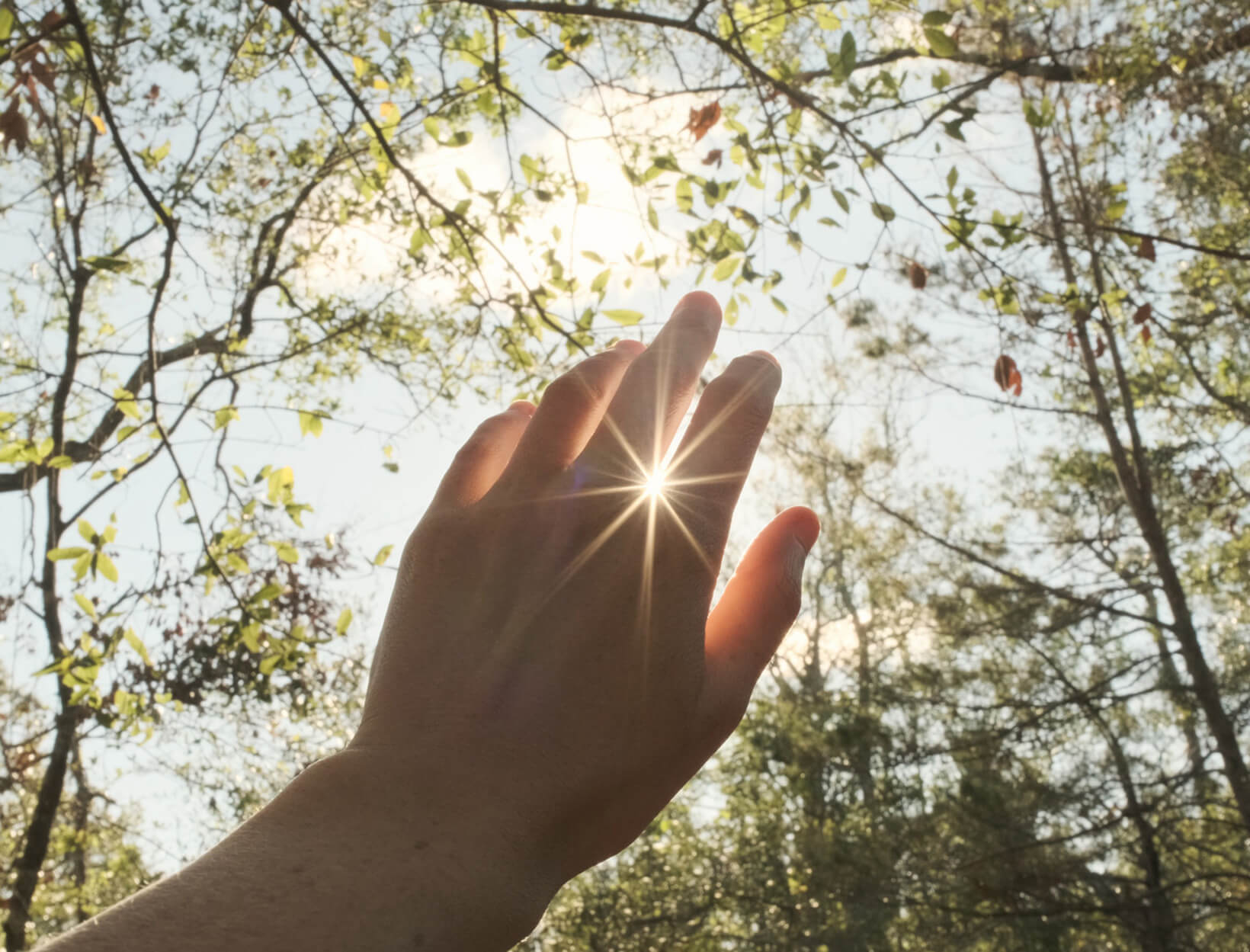A person's left hand is prominently featured, raised and stretched upwards from the lower left corner of the image, set against an outdoor wooded background. The hand’s pointer and middle fingers are artfully spread apart, allowing a beam of sunlight to filter through, aligning precisely with the camera's lens. It is daylight, with the sun positioned midway in the sky, casting a gentle, natural light. Surrounding the hand are a few trees, which frame the scene, while denser woods populate the lower portion of the background, adding to the depth and tranquility of the forest setting.